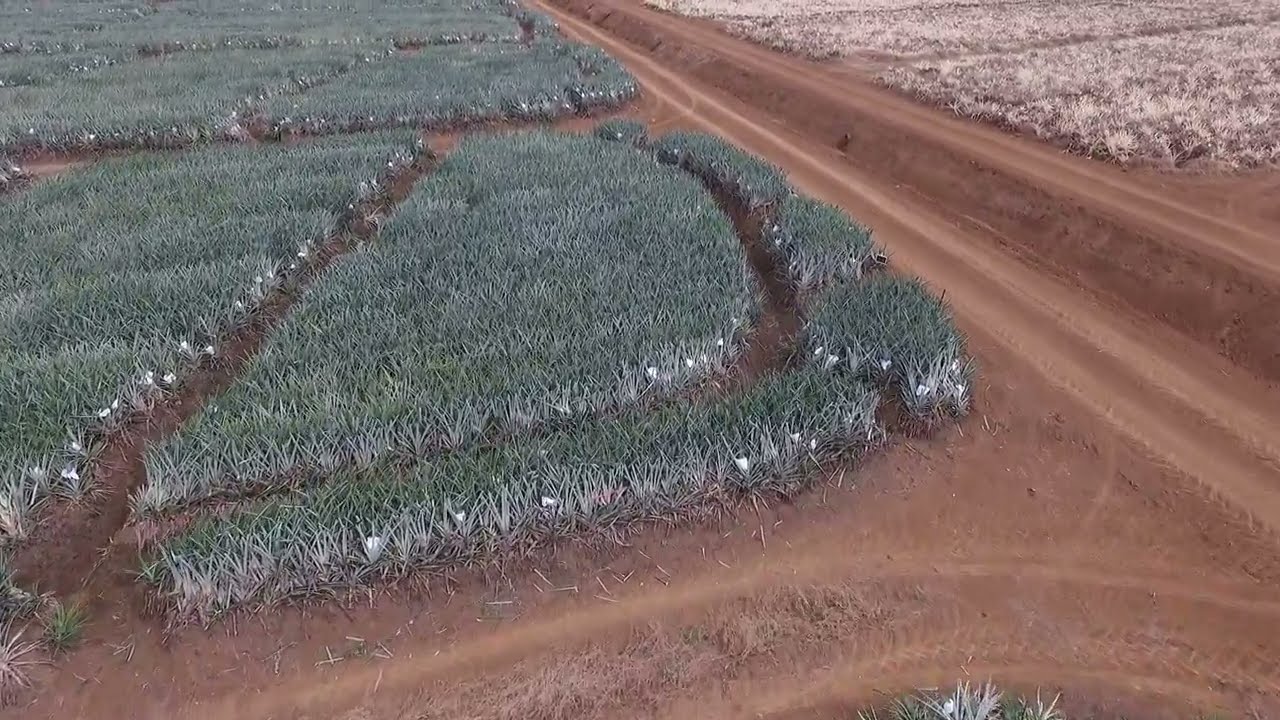The image depicts a wide expanse of a dirt field crisscrossed by multiple intertwining dirt roads, creating a network of paths heading in various directions. On the left side, there's a more prominent dirt road, almost two lanes wide, suggestive of the capacity to accommodate two cars with a median of dirt between them. To the far right, the scene transitions into a large, cultivated area filled with plants that resemble a cotton field or similarly textured crop. These plants, characterized by spiky and hard leaves, contrast with the green grass seen on the left. The grassland itself is patchy, with visible trails breaking through the verdant areas. Some parts of the grass on the right side appear frosted over, giving a white, wintry look, while the left side remains predominantly green with interspersed white patches. The entire environment is captured in daylight, providing a clear and detailed view of the varied terrain and vegetation.